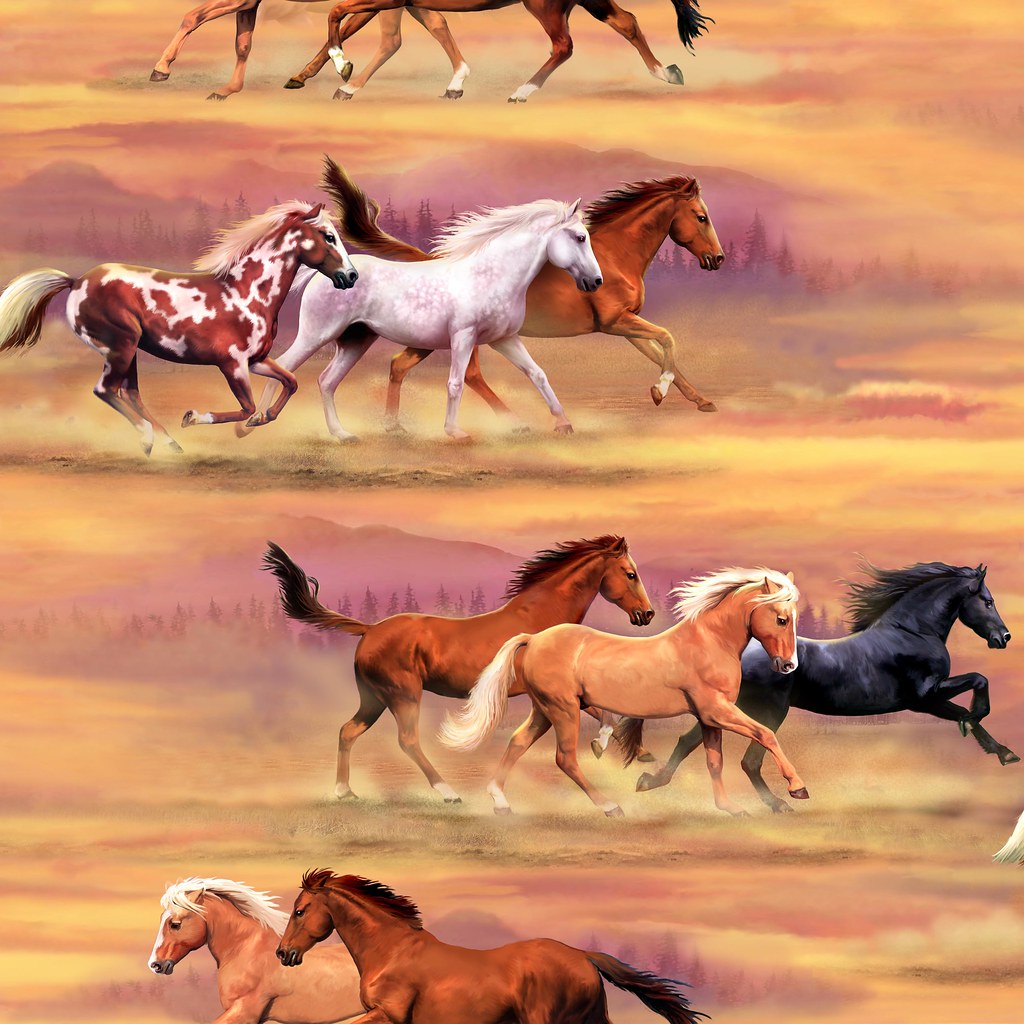The image depicts a hand-painted mural or lithograph featuring wild horses in full gallop across a vibrant, layered landscape. In the upper section, three horses—a red and white painted horse with a white mane, an all-white horse, and a brown horse with a white foot—are seen running to the right, their profiles in full display against a backdrop of misty mountains and clouds, with trees in the background and dust kicking up around them. Below, another tier of the scene shows an all-black horse, a tan horse with a white mane, a brown horse with a black mane and white feet, all galloping to the right. In the foreground, two additional horses—a brown horse with a black mane and a beige horse with a white mane—are also running. The landscape features a blend of desert and field elements, with hues of yellow, red, and orange interspersed with sporadic trees, creating a dynamic sense of movement and natural beauty as different-colored horses run in multiple directions, their powerful forms animated and energetic. The entire composition creates a rhythmic, almost repeating pattern of horses in motion, capturing the untamed spirit and freedom of wild horses.